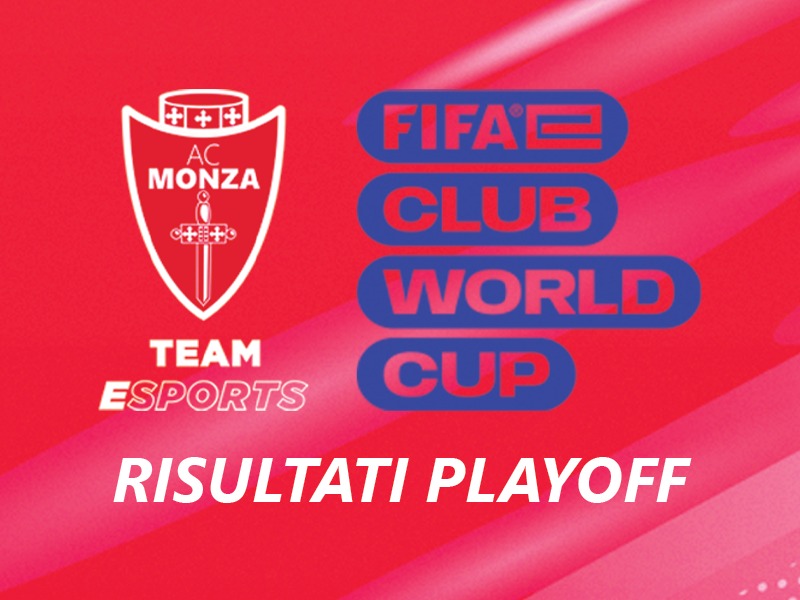This image features a red advertisement for the FIFA eClub World Cup, showcasing a dynamic background with wavy red and white patterns, transitioning from solid red in the upper left to wavy red with white streaks towards the bottom right. On the left-hand side, there's a prominent shield logo for AC Monza. The shield includes a small crown adorned with crosses at the top, a central sword symbol, and the phrase "AC Monza" above the word "eSports" in solid white, with the rest of the letters outlined in white. Beneath the shield, in white uppercase, slightly italicized letters, is the inscription "RESULTATAI PLAYOFF." Over to the right, set against the red background and incorporated within blue pill-shaped figures, the words "FIFA eClub World Cup" are displayed with each word stacked atop the other, maintaining a transparent effect that reveals the backdrop through the lettering.